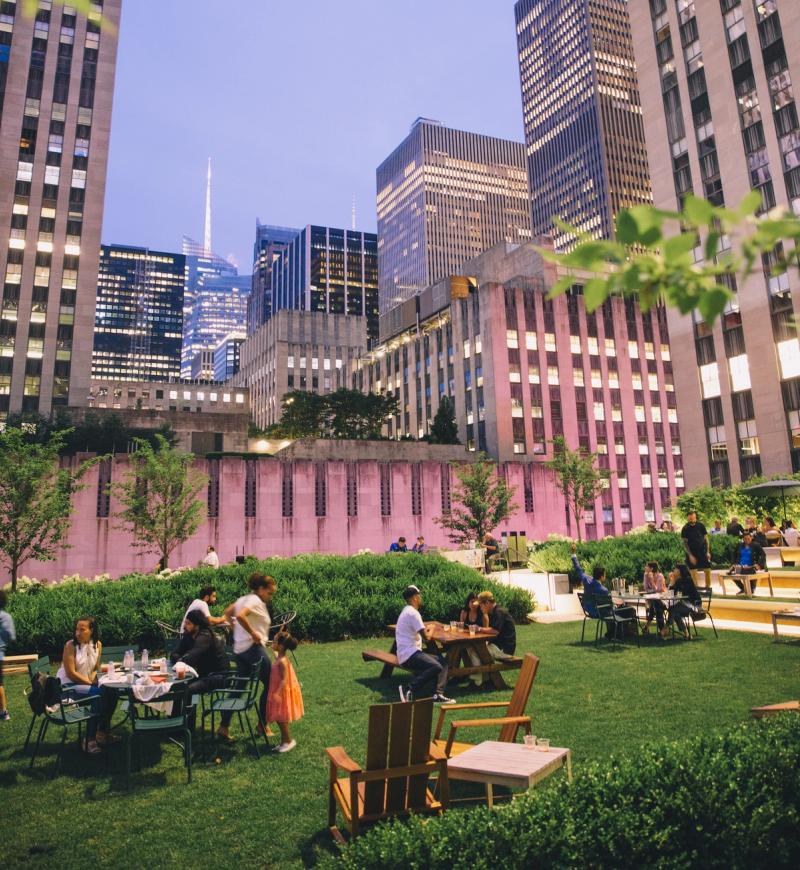The image depicts a small, park-like courtyard nestled between towering city buildings. This green space features a grassy area bordered by shrubs and scattered with various types of seating, including brown wooden chairs, wicker chairs, Adirondack chairs, green metal chairs, and picnic tables. People are gathered at these tables, either eating, talking, or drinking, with one picnic table in the background seating three individuals. Two brown wooden chairs next to a table with two empty cups can also be seen.

Adjacent to these seating arrangements, there is a concrete area and steps leading up to a multi-storied office building located in the background's right corner. On the left side and background of the photo stands an eight-story pink building, while larger, darker skyscrapers frame the scene, stretching upwards towards a partly cloudy sky with a purple hue hinting at either sunset or dusk. Dominating the skyline in the center, a tall building with a long pointed tower rises prominently above the surrounding structures, creating a striking urban backdrop for this serene courtyard.